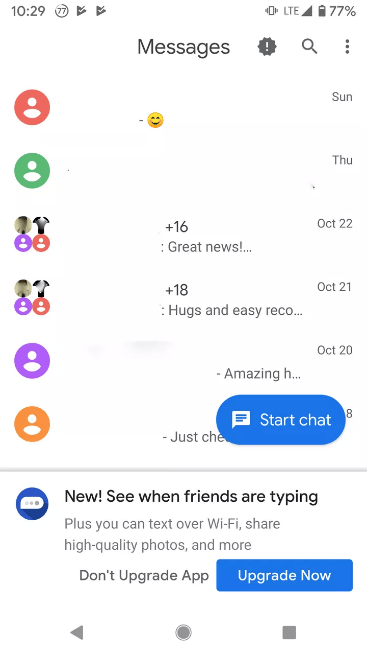The image is a screenshot taken on a mobile device with a time stamp of 10:29 displayed at the top left corner. The background is predominantly white and showcases various icons and notifications. On the top right corner, indicators show an LTE connection and a battery level at approximately 77%, although it is not currently charging.

Below this, there are messaging notifications. The first message features a red circle with a white user icon depicting a smiling face, sent on Sunday. The second message is from a user with a green background, also with a white icon, sent on Thursday. There is an indication of a group chat involving four people, identified by their colored icons: a purple background, a red background, and two additional participants.

Noteworthy details within the chat include:
- A message stating "plus 16, great news" sent on October 22nd.
- Another message saying "plus 18, hugs and easy reco..." sent on October 21st.
- A partial message reading "amazing, H..." dated October 20th.

Additionally, a prominent blue button labeled "Start Chat" is visible. The bottom of the screen features a new notification highlighting that users can see when friends are typing, text over Wi-Fi, share high-quality photos, and more.